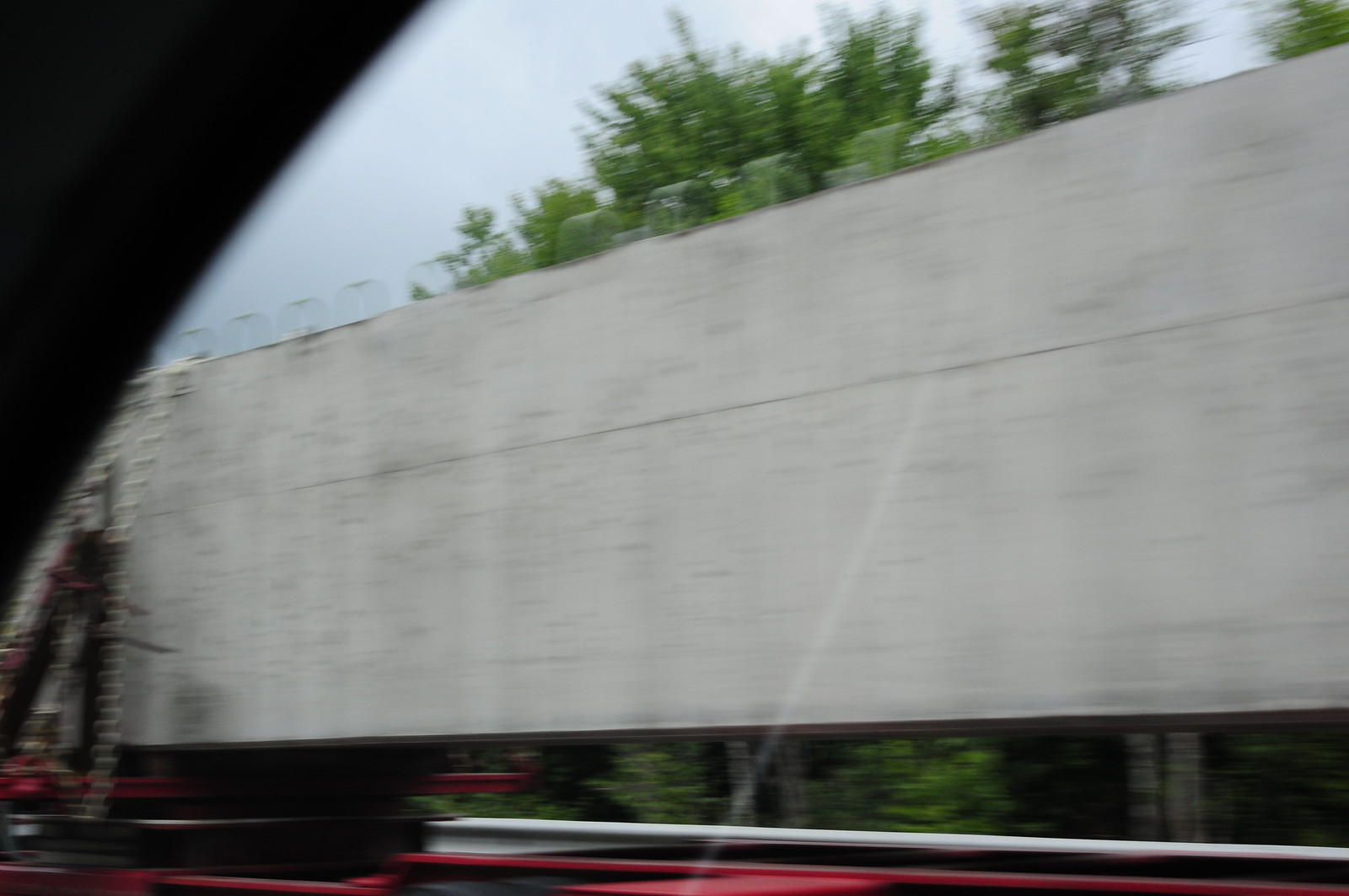The photograph presents a very blurred scene reminiscent of a view from the backseat of a moving car. On the left side, a black triangular shape suggests the perspective from a car window, framing the image. Dominating the center is a tan, rectangular shape that could be an 18-wheeler or a lengthy wall, with a streak running down the middle that enhances the sensation of looking through glass. Below the tan structure, a streak of red adds a splash of color. In the background, trees peek out both beneath and above the tan object, set against a backdrop of blue sky. Atop the tan structure, small, indistinct wire-like shapes are visible. The overall effect is one of rapid motion, with the entire scene gliding past the viewer in a blur.